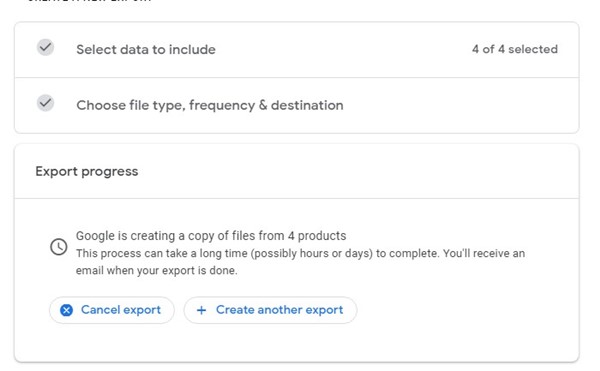The image is a horizontally oriented screenshot with a predominantly white background featuring instructions and status updates related to data export from Google. 

- In the top-left corner, there is a light gray circle with a darker gray check mark inside it, next to the text "Select data to include" in gray font.
- Towards the top-right corner, the text "4 of 4 selected" is displayed.
- This section is enclosed by a light gray border.

Below this, another section has a similar light gray circle with a darker gray check mark and the text "Choose file type, frequency, and destination."

Separated by a small space, another rectangular section contains the bolded black text "Export progress."

Further down, a larger horizontal rectangle displays an informational message: "Google is creating a copy of files from 4 products. This process can take a long time (possibly hours or days) to complete. You'll receive an email when your export is done."

At the bottom of the page, there are two outlined ovals with a white background and a gray border:
- The oval on the left has a colored-in circle with a white ‘X’ and the text "Cancel export."
- The oval on the right has a plus sign and the text "Create another export."